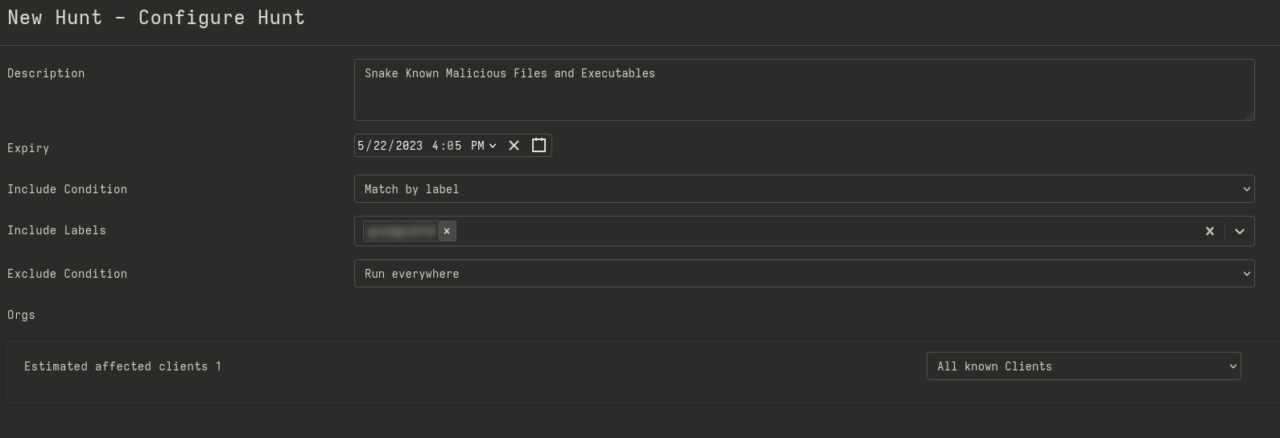This image is a screenshot displaying a configuration interface for a hunting tool. The picture is rectangular with a black background, featuring predominantly white text. 

At the top left corner, there is the heading "New Hunt - Configure Hunt." Beneath this heading, a thin, pale white horizontal line runs almost across the entire width of the image.

Below this line, on the left side in a smaller white font, the word "Description" can be seen. Next to "Description," although a bit faint, the typed words are present, which seem to read something like "Snake" and "Known Malicious Files," though this is not entirely clear due to the faintness.

This section is enclosed within a rectangular box. Underneath this box is the word "Expiry," alongside another rectangular box that contains a date. 

Following this, the words "Include Condition" appear next to yet another rectangular box that seems to indicate "Match by Label." Below this, the phrase "Include Labels" is displayed. 

Continuing downward, the text reads "Exclude Condition," with another word situated beneath it.